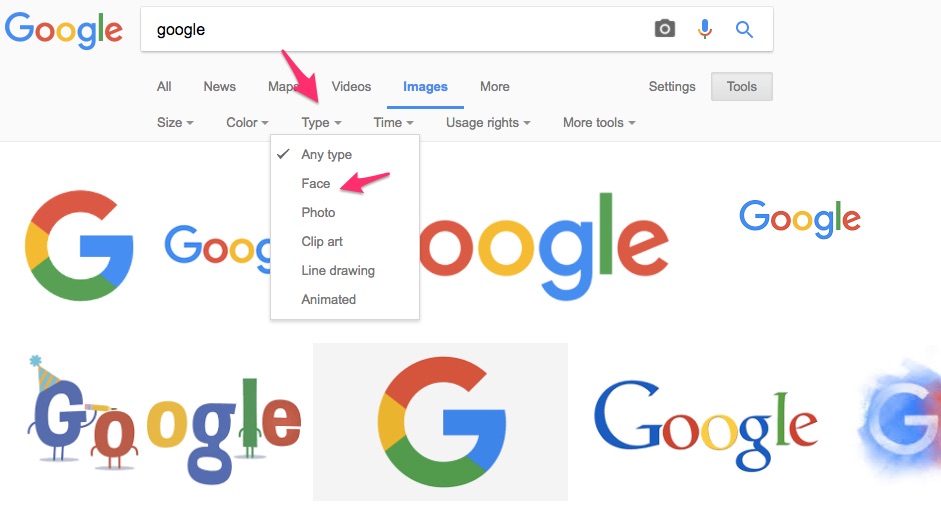The image displays a colorful, multi-layered Google-themed artwork. The main highlighted feature is the iconic "G" logo, adorned with a festive party hat and streamer, positioned prominently within a larger composition. The artwork is organized within a square, and the colors reflect Google's signature palette.

In the upper portion of the square, there are several instances of the word "Google" in various sizes. The most prominent "G" stands out with a party hat and streamer, adding a celebratory touch. Another "G" is seen on a gray square, providing contrast to the white background of the primary square. 

There's also a third "G" with a background that appears to have a blue and pink chalk smear slightly to the right, adding a playful texture to the backdrop. At the very top of the image, "Google" is repeated alongside a search bar featuring a camera, microphone, and magnifying glass icons, suggesting a search interface.

Below the search bar, there are filter options including "Size," "Color," "Type," "Time," "Usage Rights," and "More Tools." A red arrow points to "Type," where another filter menu shows a checked option for "Any type" with additional options like "Face" (highlighted by another red arrow), "Photo," "Clip Art," "Line Drawing," and "Animated."

To the side, the interface displays "Settings" and "Tools" highlighted on a gray rectangle. At the top navigation bar, the tabs "All," "News," "Maps," "Videos," and "Images" are visible, with "Images" highlighted in blue to indicate the current selection. The "More" option indicates further choices available to the user.

In summary, the image intricately combines various elements of Google's branding and its search interface, enhanced with playful, celebratory details, and navigational hints that suggest an in-depth usage context.